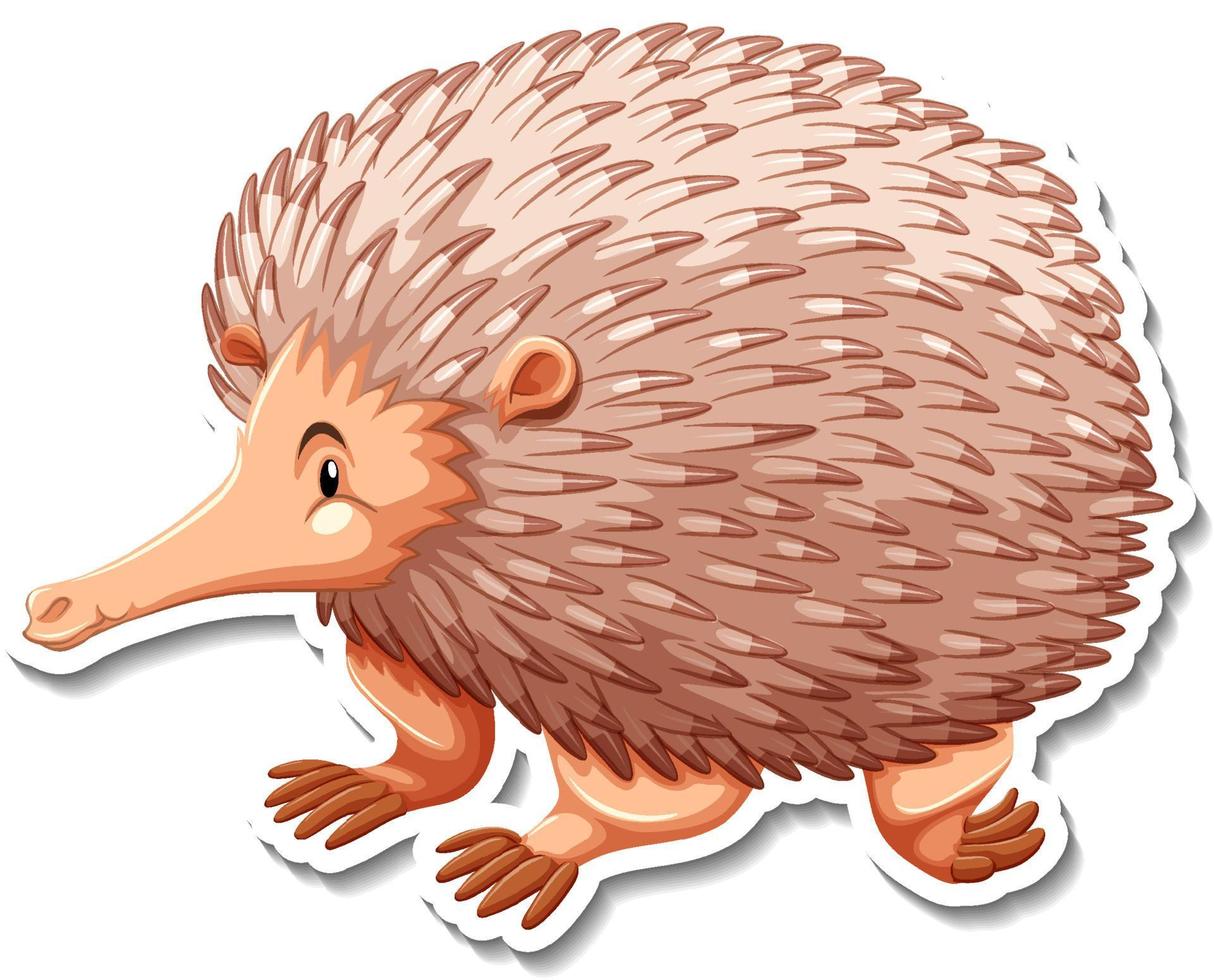This is a detailed, color image of a cartoon porcupine, which has been either drawn or painted, and potentially cut out and pasted onto a white background to give a 3D effect. Its body is shaped like a large bowl, showcasing a gradient from dark brown at the top to an even darker shade towards the bottom. The porcupine is adorned with light pink spikes that have brown tips, all laying backwards. The face, positioned on the left side, features a long, bent nose, a single black oval eye under an arched black eyebrow, and a light cream-colored skin tone with a white circle beneath the eye. One visible ear adds to its expressive look. It has three visible legs, each with toes: the front legs have long, forward-facing toes, dark brown in color, and one of the back legs has toes bent inward, facing right. The entire figure is outlined by a distinct white border, enhancing its cutout appearance against the white background.